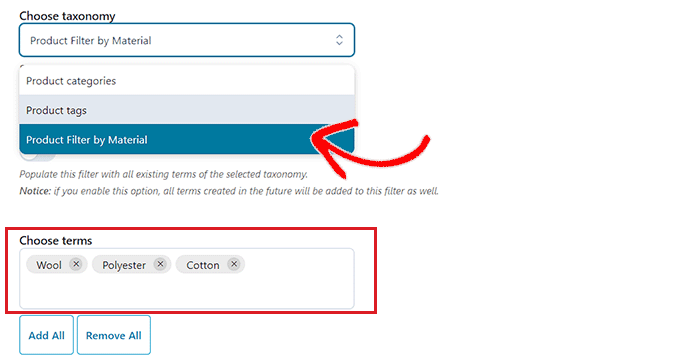This image captures a screenshot of a digital form with a white background, annotated with red markings for clarity. In the upper left-hand corner, the heading reads "Choose Taxonomy," spelled out as t-a-x-o-n-o-m-y. Below this, there is a dropdown menu labeled "Product Filter by Material," complete with up and down arrows for navigation.

On the subsequent row, the form lists "Product Categories," "Product Tags," and a repeated "Product Filter by Material," the last of which is highlighted with a teal background. A handwritten red arrow points directly to this row, emphasizing the "Product Filter by Material" section.

Beneath this, instructional text explains: "Populate this filter with all existing terms of the selected taxonomy. Notice if you enable this option all terms created in the future will be added to this filter as well."

The next part of the form, professionally bordered in red by the annotator, is titled "Choose Terms." In this specified area, the user has typed in potential terms: "wool," "polyester," and "cotton."

In the lower left-hand corner of the form, two buttons are visible: the first reads "Add All," and the second reads "Remove All." The form currently indicates the selection of the taxonomy and the product filter by material, with specific material terms chosen as "wool," "polyester," and "cotton." It is implied that the next logical step would be to use the "Add All" button, although this particular action is not marked with an arrow.